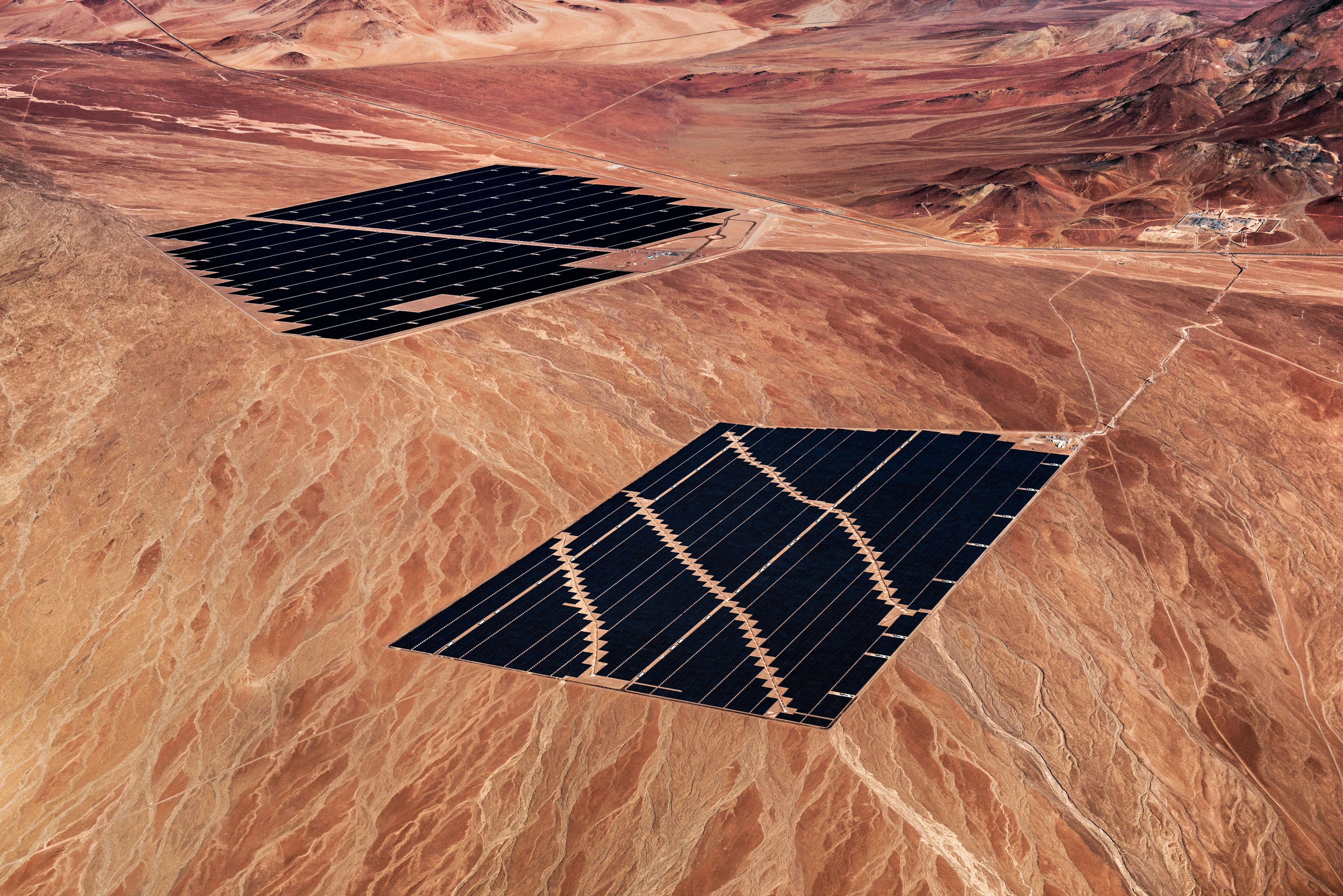The image depicts a barren, desert-like landscape with a striking reddish-orange and light yellowish veined pattern traversing the dried dirt. Two black rectangular panels, resembling solar panels, lie prominently on the ground amidst the rough, cracked terrain. The background features ridges and distant mountains, hinting at varied elevations. Interwoven through the scene are peculiar squiggles and yellow jagged lines. Adding to the surreal atmosphere are elements that evoke a sense of Mars-like isolation, enhancing the overall conceptual nature of this painting. Scattered buildings are linked by a trail, and a road cuts through the image, hinting at some semblance of human presence amidst the desolate environment.